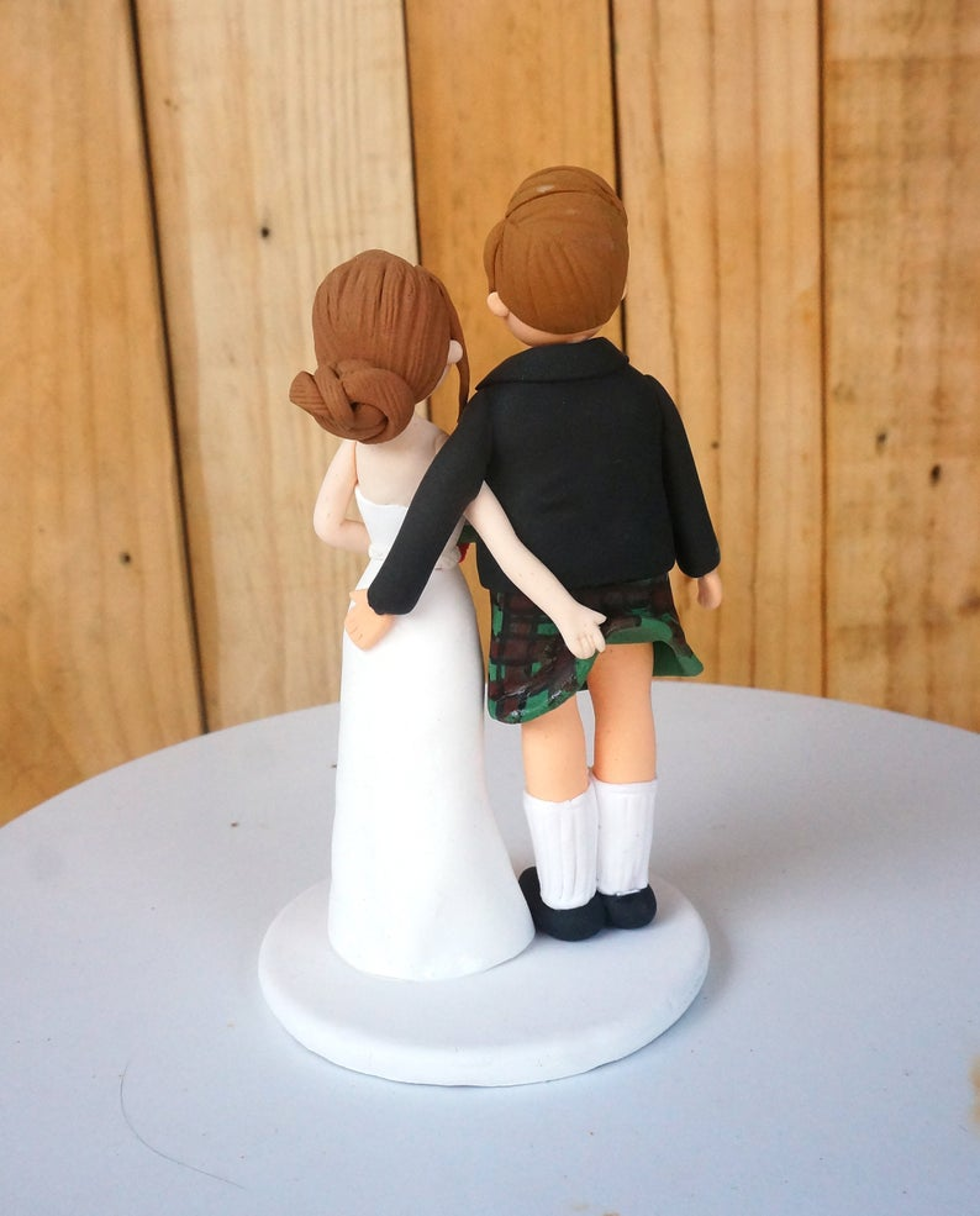This photograph showcases a humorous wedding cake topper featuring two figurines in a playful pose. The couple is seen from the back, with the woman on the left and the man on the right. The woman is wearing a strapless, full-length, conventional white wedding gown, and has her brown hair tied in a bun. The man is dressed in a black suit jacket paired with a green and brown Scottish kilt, white socks, and black shoes. The woman amusingly lifts the man's kilt with her right hand, while the man has his left hand resting on her rear end, adding a comical touch to the scene. Both figurines have brown hair and are mounted on a circular white platform, which is placed on a larger circular surface, likely a table. The background is a wooden wall, enhancing the cozy and rustic setting of this whimsical tableau.